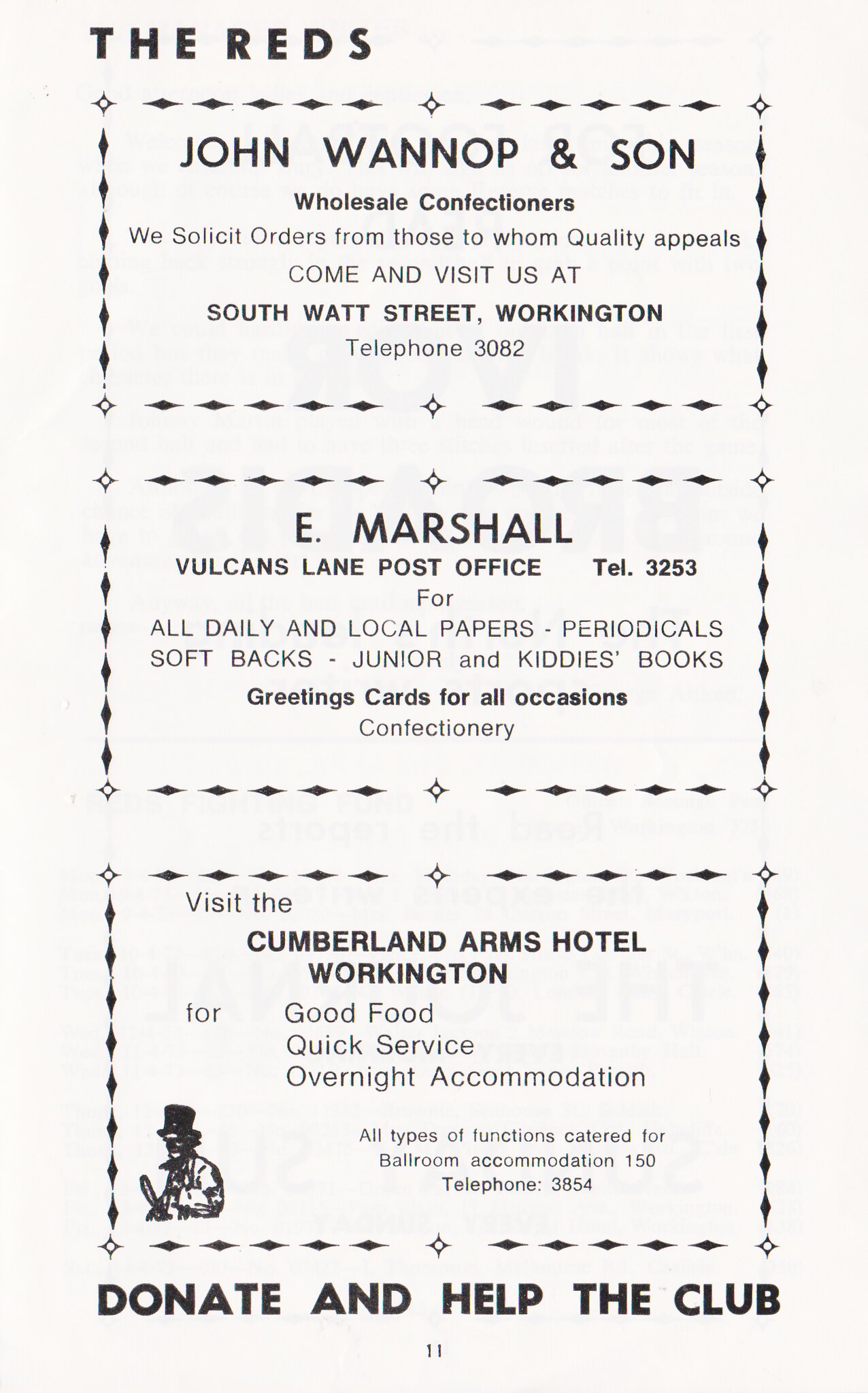The image depicts a pink piece of paper, likely a page from a larger pamphlet or book, labeled as "page eleven." At the top left corner, it prominently displays "The Reds," suggesting it may be referring to a club or organization by that name. The central message, "donate and help the club," appears at the bottom in black text, emphasizing a call for support.

Three black-and-white rectangular advertisements are featured on the page, reflecting an old-time aesthetic with minimal graphics. The first ad at the top is for "John Wanup and Son," who are wholesale confectioners that invite orders from quality-conscious customers. The second ad is for "E. Marshall" of Vulcans Lane Post Office, offering daily and local papers, periodicals, softbacks, junior and children's books, and greeting cards for all occasions. The final ad promotes the "Cumberland Arms Hotel" in Workington, highlighting good food, quick service, and overnight accommodations.

Overall, the page presents a blend of advertisements and a fundraising appeal, capturing a vintage snapshot of community commerce and support.